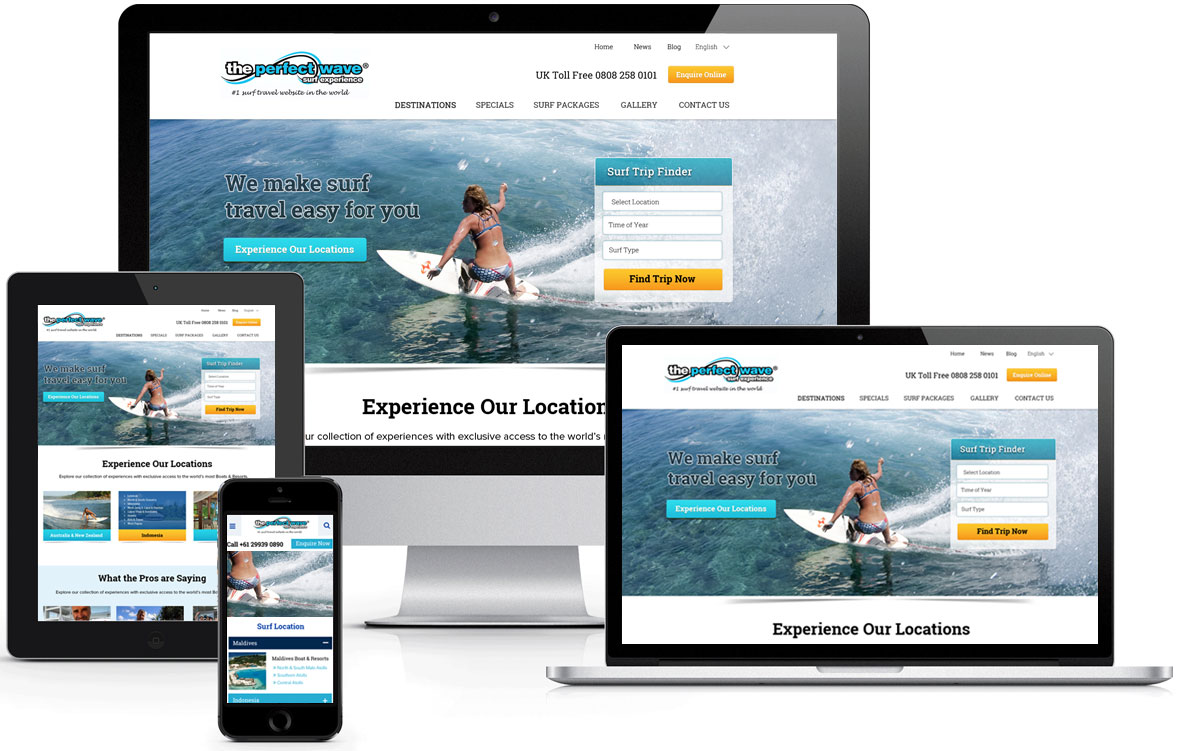A promotional image from the website "The Perfect Wave" showcases the accessibility and versatility of their platform across multiple devices, including a mobile phone (black iPhone), a tablet, a laptop, and a desktop computer. The company’s tagline, "We make surf travel easy for you," is prominently displayed, emphasizing their focus on simplifying surf travel arrangements.

The image features a vibrant action shot of a woman joyfully surfing on a large, clear blue wave, capturing the essence of exhilarating surf adventures. The website interface, visible on the devices, offers various services and features including destination guides, special offers, and comprehensive surf trip packages. Users are invited to explore locations in the UK and beyond, with the added convenience of a UK toll-free number for personalized assistance.

Additionally, the site includes a "Surf Trip Finder" tool, where users can input their preferences and hit an orange button to discover tailored surf trips. Other navigational elements highlighted in the image are the gallery, contact us page, and detailed sections for different travel packages, aimed at enhancing the user’s browsing and booking experience.